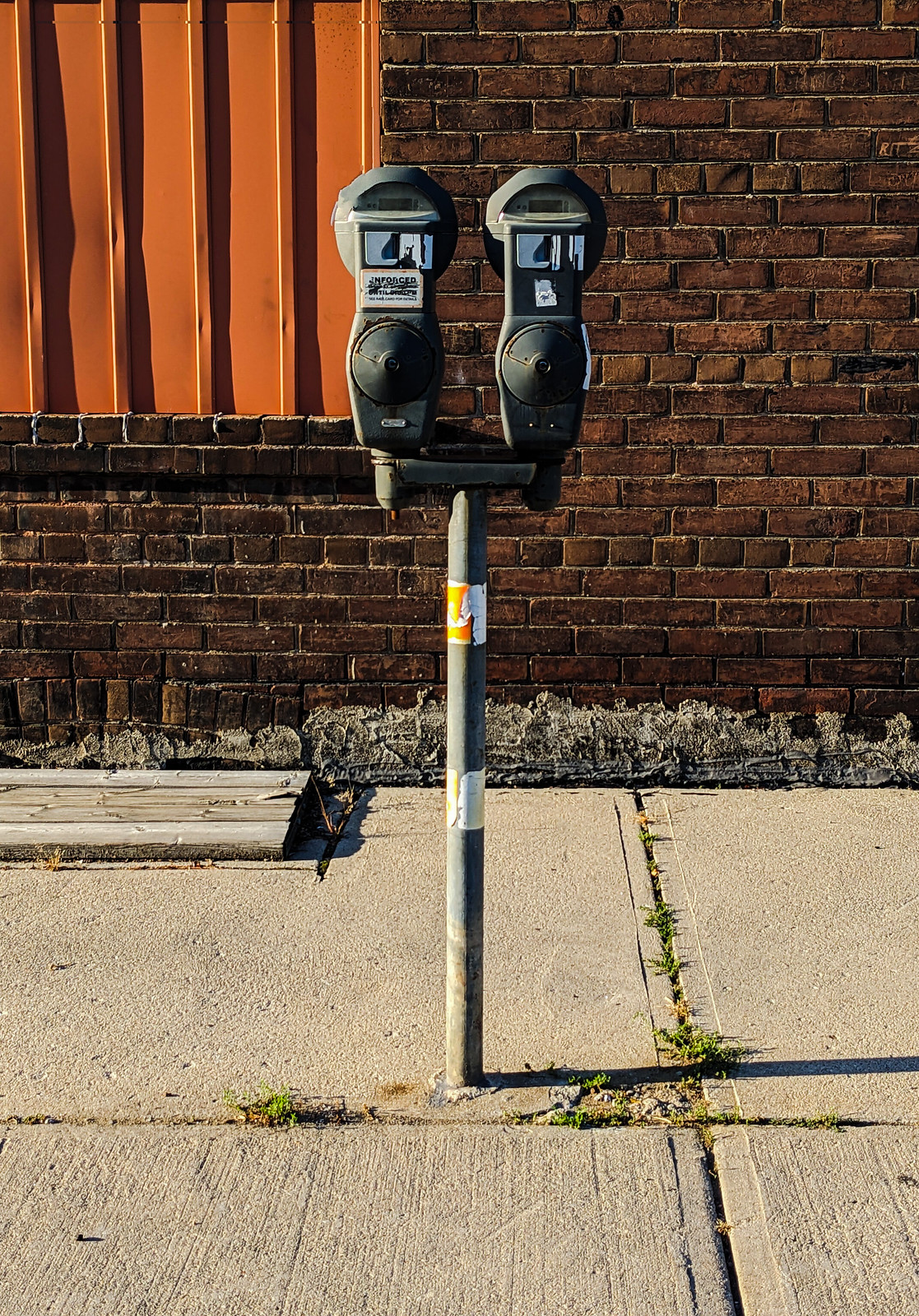This colour photograph captures a typical coin-operated parking meter with two heads, mounted on a straight pole that is cemented into a sidewalk. The parking meter, which looks quite old and possibly antique, features peeling stickers — a partial yellow and white sticker near the top and a white one halfway down. Each of the two gray heads on the meter has circular slots for coins and windows displaying the remaining parking time. The pole is firmly set in a cracked cement sidewalk, with some weeds and dead grass growing between the cracks.

In the background, there is a brown brick wall, which has a spattering of spackling or mortar at its base. A window cut into the wall features vertical orange blinds and possibly metal bars. To the back left of the scene, there is a wooden, flat door leading to a basement or sub-level, with horizontal planks visible. The overall setting provides a sense of urban decay, with small details hinting at the passage of time and wear.